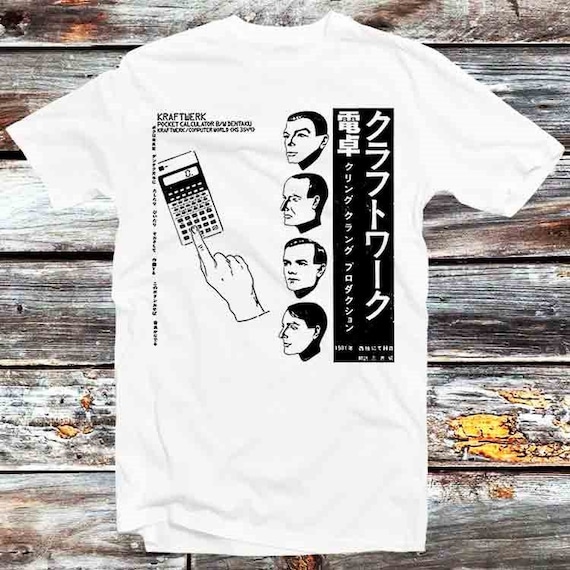The image is of a white short-sleeved t-shirt set against a background of weathered wooden planks in various shades of brown, gray, white, and yellow. The t-shirt features a detailed black screen-printed design. On the left side, a disembodied hand with an index finger is seen pressing a zeroed-out old-fashioned calculator. Above the calculator, the text reads, "Kraftwerk Pocket Calculator," though some additional text beneath it is too blurry to decipher clearly. To the right of the calculator are four pencil-sketch profiles of men with short hair, seemingly from the band Kraftwerk, given their blank expressions and distinct positioning, with slight variations in the direction they are facing. On the far right, a vertical black banner with Japanese characters runs alongside the profiles. The text and design elements evoke a nostalgic sense, possibly referencing an original design from the 1980s.